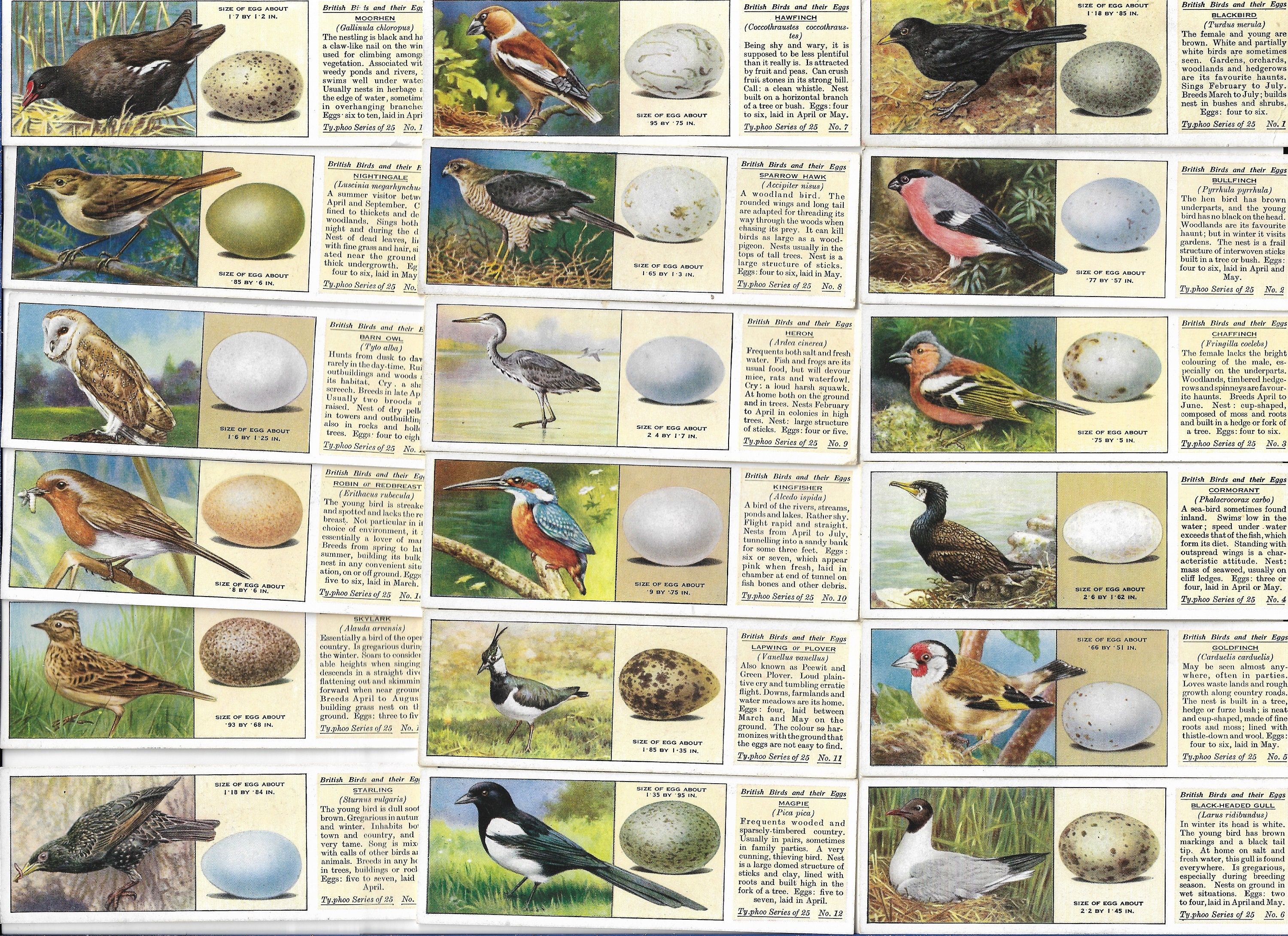This is a highly detailed, hand-drawn diagram likely from a textbook or educational poster, showcasing 18 various bird species and their corresponding eggs. The birds are arranged in three columns, each accompanied by their respective eggs and descriptive text, although the text is too small to read clearly. The background is beige, unifying the earthy tones throughout the illustration.

The first column features:

1. A brown bird with white accents and a red beak, paired with a white egg with brown dots.
2. An olive bird with a white underbody and an olive-green egg.
3. A light brown owl with a white underbody, matched with a plain white egg.
4. A golden-brown finch with a red neck, black beak, and white underbody, with a beige egg dotted in brown.
5. A primarily brown finch with a lighter underbody and dark brown stripes, accompanied by a brown egg with black dots.
6. A finch with a small tan beak and a black-and-white striped body with a light brown underbody, and a white egg.

The second column includes:

1. A brown bird with white and black markings, with an egg featuring black swirls.
2. A bird with brown stripes on a beige body and black wings, paired with an egg speckled in brown.
3. A gray and white swan with a striking blue egg.
4. A bird with blue feathers, a blue head, an orange body, and a white egg.
5. An olive and white bird with a brown egg dotted in black.
6. A blue and black bird with a white body and a green egg.

The third column profiles:

1. A black bird with a black egg marked with white spots.
2. A red and gray bird with black feathers and a white egg.
3. A multicolored bird with shades of orange, gray, and olive, alongside a white egg with olive spots.
4. A green and brown duck with a white egg.
5. A primarily brown multicolored bird with yellow and black accents on its wings and a white egg.
6. A gray and white bird with a red or brown head, paired with a brown egg speckled with darker brown spots.

The vibrant yet natural color palette used in the illustrations—ranging from browns and beiges to more vivid reds and blues—conveys the diverse beauty of each bird species and their eggs. The overall layout and depiction of details provide an educational and visually appealing source of information for students or bird enthusiasts.